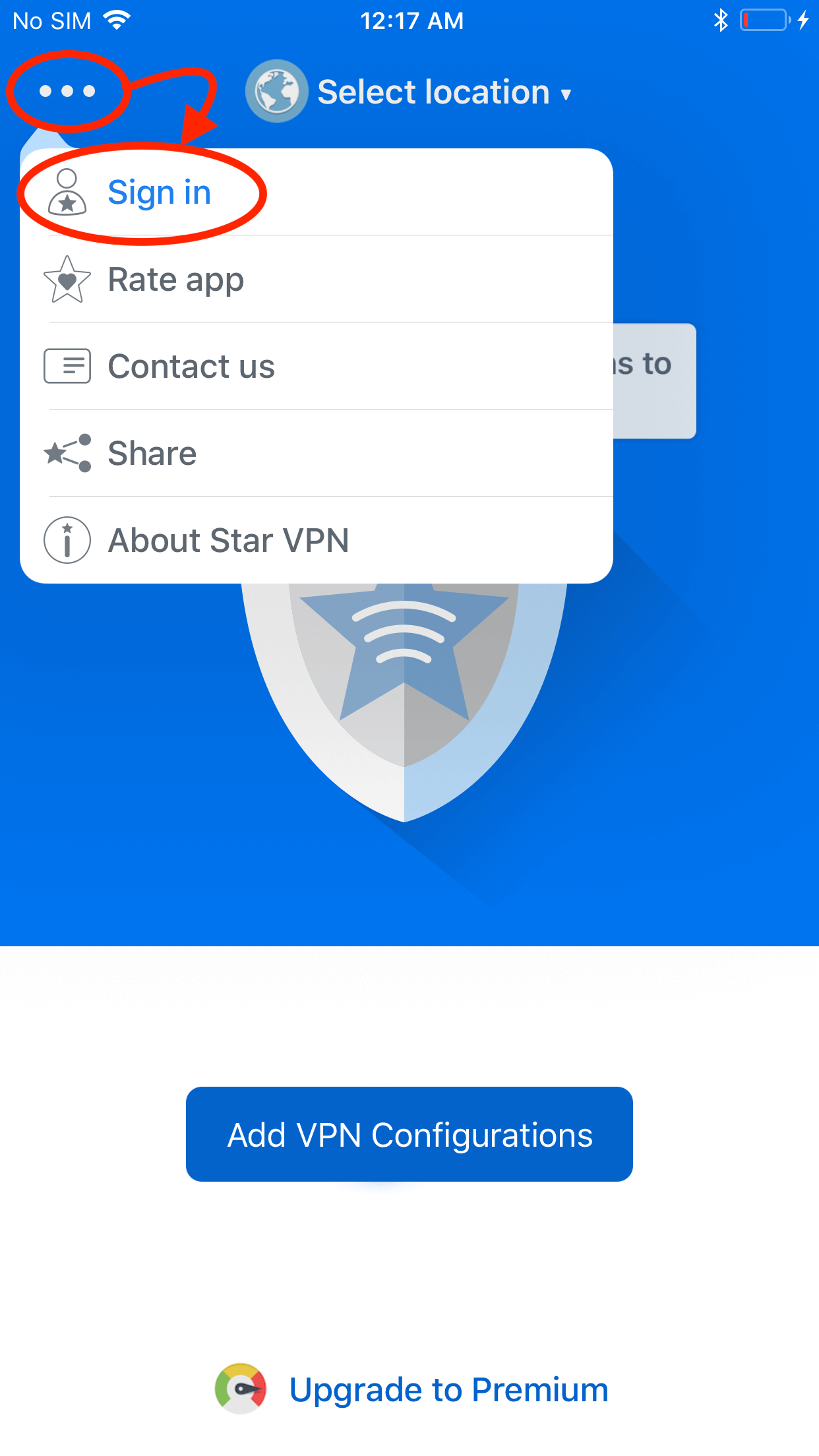This screenshot appears to be taken from a mobile device showcasing an app, presumably a VPN service, with instructions on how to log in. The interface has 1270nm displayed prominently at the top. Notably, the device's status bar shows critical details: the battery level on the right is very low, indicated by a small red segment, and "No SIM" is displayed on the left.

The app screen features a royal blue background, with a "Select Location" option accompanied by a small grey globe icon. To the left of this, there are three horizontal white dots encased in a red oval, with a small arrow transitioning out of the oval, highlighting the word "Sign In" along with a dropdown menu.

This dropdown menu contains five items:
1. **Sign In** - represented by a person icon with a grey star.
2. **Rate App** - denoted by a star intertwined with a heart.
3. **Contact Us** - illustrated with an icon resembling a business card.
4. **Share** - marked by a grey star emitting two lines ending in circles.
5. **About STAR VPN** - symbolized by a circle encompassing an eye.

Additionally, a partially visible shield icon with a star can be seen within the blue background. Toward the bottom of the screenshot, there is a white section followed by a blue rectangular button with "Add VPN Configurations" written in white text. At the very bottom, in blue text, it reads "Upgrade to Premium."